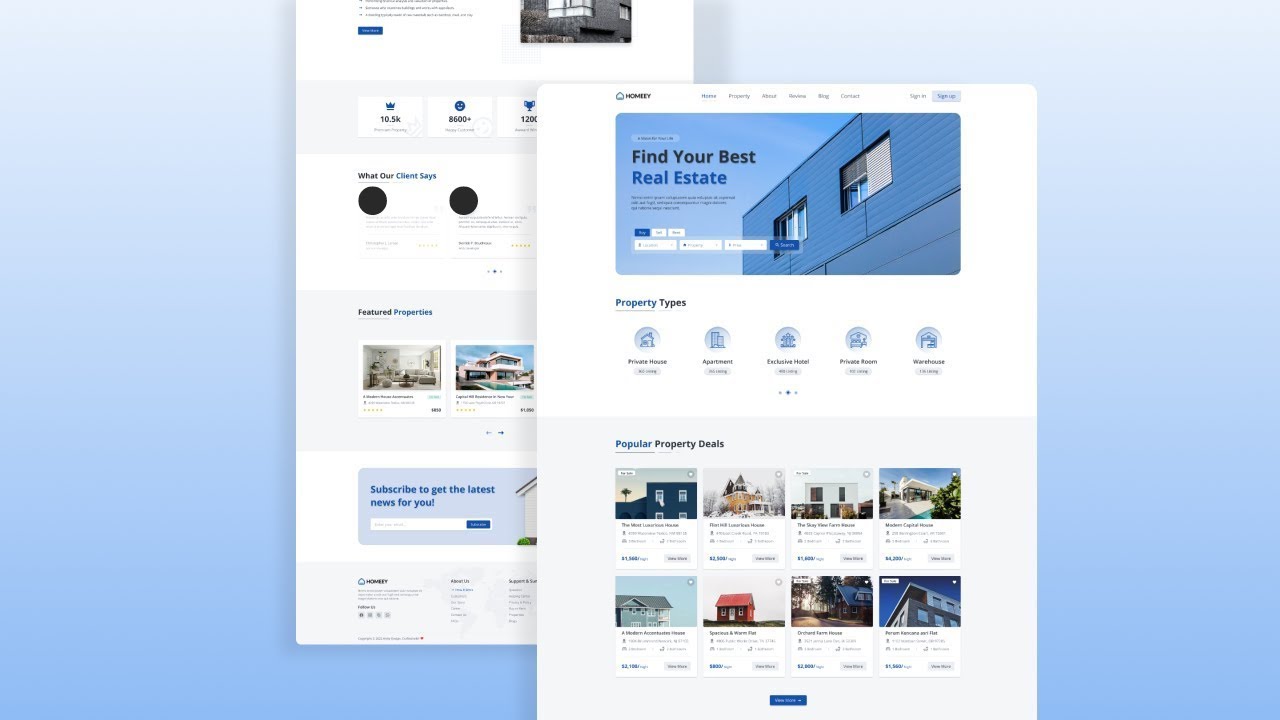The image features a blue background with two overlapping real estate webpages. The webpage in the foreground belongs to 'Homee'—spelled H-O-M-E-E-Y—which is prominently displayed alongside a small house icon. The top navigation bar includes categories such as "Homes," "Property," "About," "Blogs," "Contact," and "Reviews." The 'Homes' section is currently selected, displaying the tagline "Find Your Best Real Estate" beneath an image of a residential building. 

This page also features interactive elements: multiple text boxes, buttons, and drop-down menus for refining property searches. Users can filter property types by selecting options like private house, apartment, exclusive hotel, private room, or warehouse. Additionally, it showcases "Popular Property Deals," listing eight different properties with various prices and characteristics.

In the background, another section of the Homee site is slightly visible. This section highlights some numerical statistics, including "10.5k," "80,000," and "8,600+," the context of which is unclear. It also features a subscription form inviting users to "Subscribe to the Latest News" and a testimonial section titled "What Our Client Says," which presumably contains client reviews and feedback about the services offered by the website. The overall theme suggests this is a comprehensive real estate platform designed to assist users in finding diverse property options.